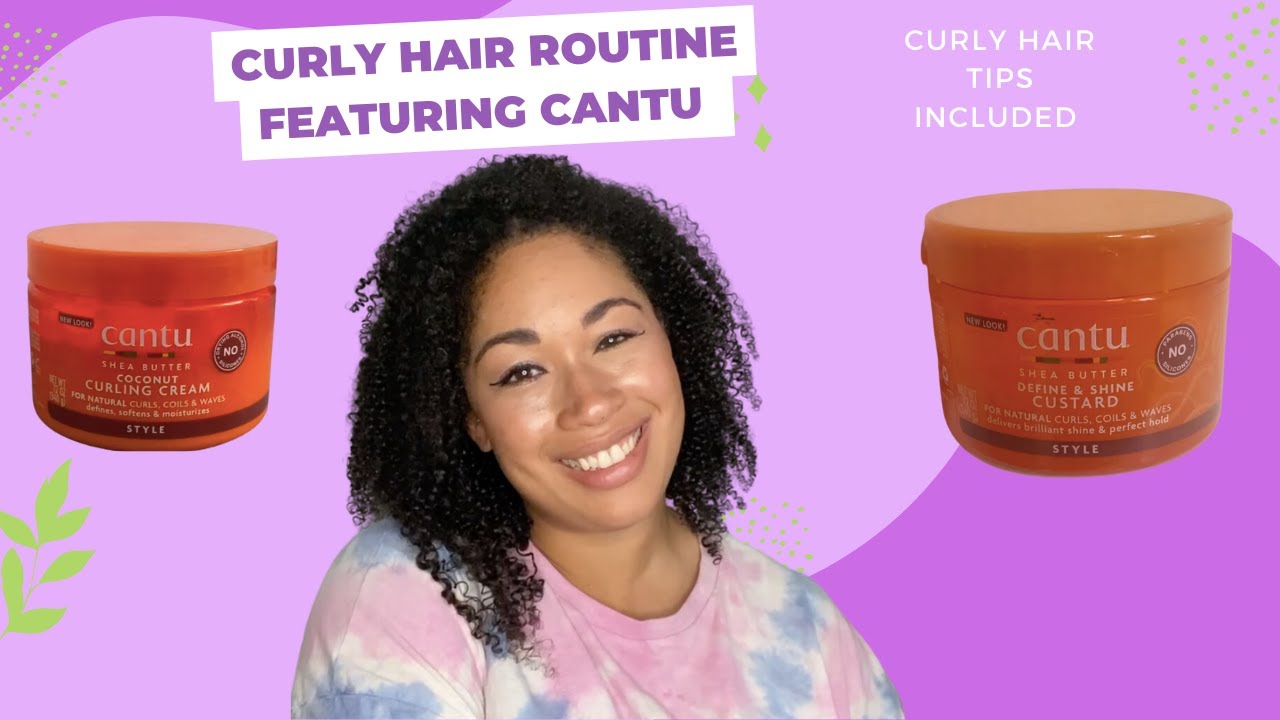The image is a vibrant, full-color promotional ad for a hair product, formatted in a horizontal rectangle. The background features varying shades of purple, with deeper tones in the corners and a lighter lavender sweeping diagonally through the middle. Centered in the image is a smiling African American woman, captured from the torso up. She boasts dark, curly hair and wears a striking pink, blue, and white tie-dye t-shirt. Her head is gently tilted to the left, enhancing her warm expression. Positioned in the top left corner is a white banner with purple text stating, "Curly Hair Routine featuring Cantu," and directly opposite, in the upper right corner, another white banner reads, "Curly Hair Tips Included." On either side of the woman are two orange Cantu containers: one labeled "Shea Butter Coconut Curling Cream," and the other, "Shea Butter Define and Shine Custard." In the bottom left corner, green leaves subtly peek into the frame, adding a natural touch to the visually appealing advertisement.